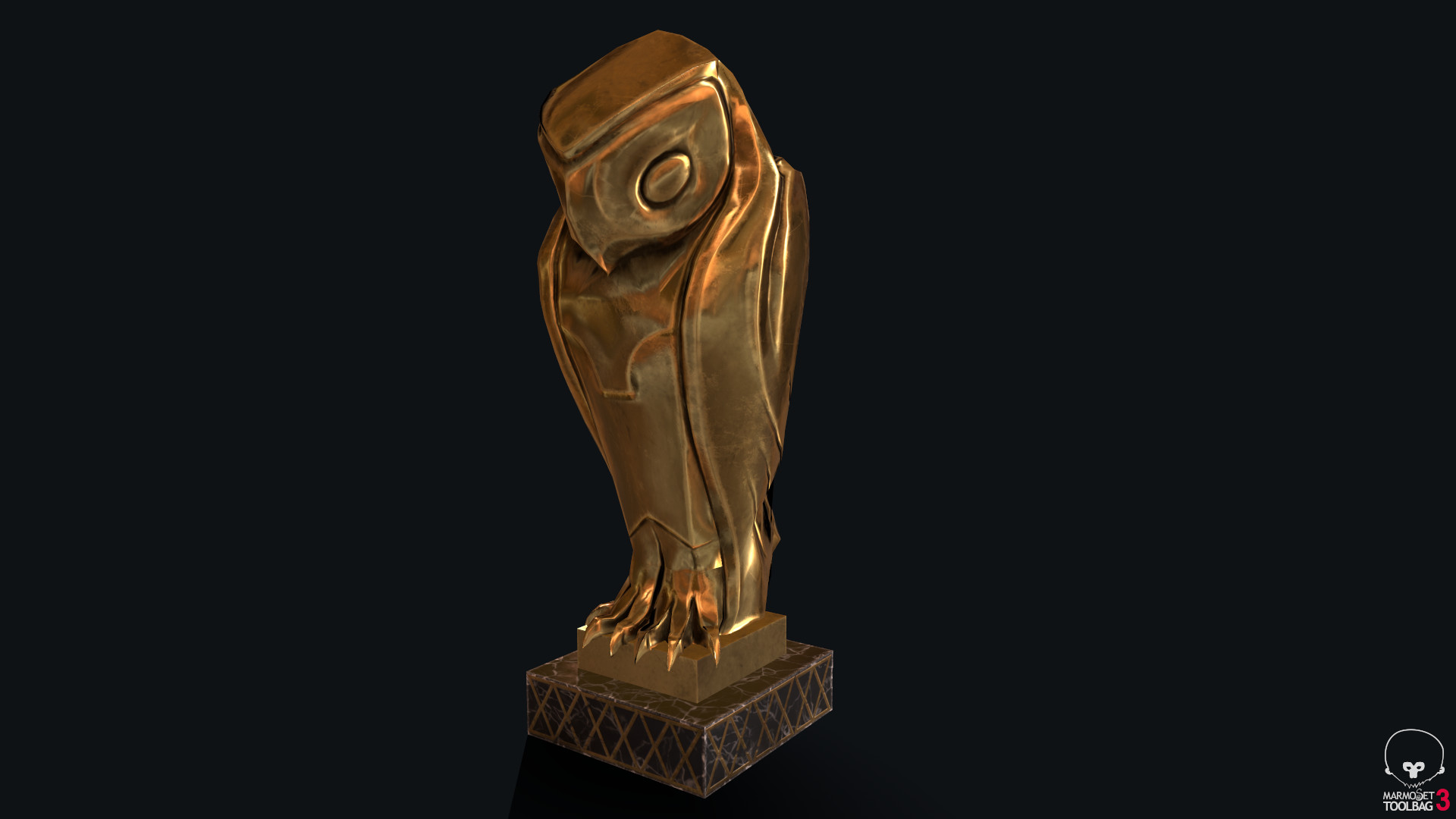This image depicts a detailed and stylized statue of a bird, possibly an owl or falcon, crafted from gold or bronze, set against a solid black background. The bird stands majestically on a layered pedestal. The lower pedestal is a darker gold or brown color, marked with a distinct 'X' pattern and likely made of dark gray marble. Atop this is a smaller pedestal, matching the bird in its golden hue. The bird itself, with its streamlined and angular design, has minimal yet deliberate details: three-pronged talons grasp the pedestal, wings are tucked closely by its sides, and its head, which has a carved-out eye and a sharp, short beak, faces downward. Intriguingly, the bird's body, reminiscent of a vase shape, appears to wear a stylized "vest" formed by its smooth, clean lines. To the bottom right of the image, there's a notable red inscription that reads "Marmoset Toolbag 3."